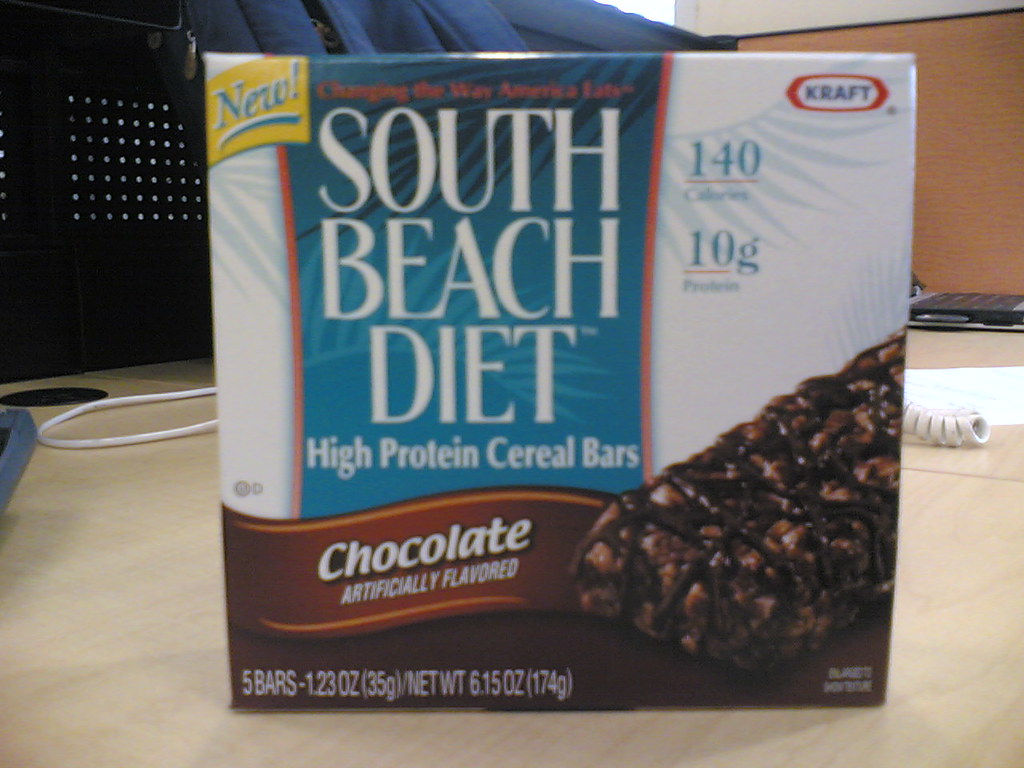The image is a close-up, slightly blurry photograph of a box of South Beach Diet High-Protein Cereal Bars, prominently displayed against a wood desk surface with a laptop and phone cable visible in the background. The box is facing forward, showcasing all the critical details on its front. 

At the top left corner, a yellow background highlights the word "NEW" in white text. Directly below, a brown ribbon states "Chocolate Artificially Flavored" in white text. The predominant teal background of the box also features delicate fern or palm leaf designs. The box emphasizes its high-protein content with "140 calories" and "10 grams of protein" clearly printed on the front. In the middle of the box, the slogan "Changing the way America eats" is displayed in red text followed by "South Beach Diet High-Protein Cereal Bars" in white text. 

Toward the bottom, the right third of the box features an image of the cereal bar at a 45-degree angle, showcasing its chocolate drizzle. The bottom left notes "5 bars, 1.23 oz (35g)" with a total net weight of "6.15 oz (174g)." At the very top right, the word "craft" is visible, completing the detailed front view of this product's packaging. The background scenery suggests it is daytime, as indicated by light coming through an unseen window.